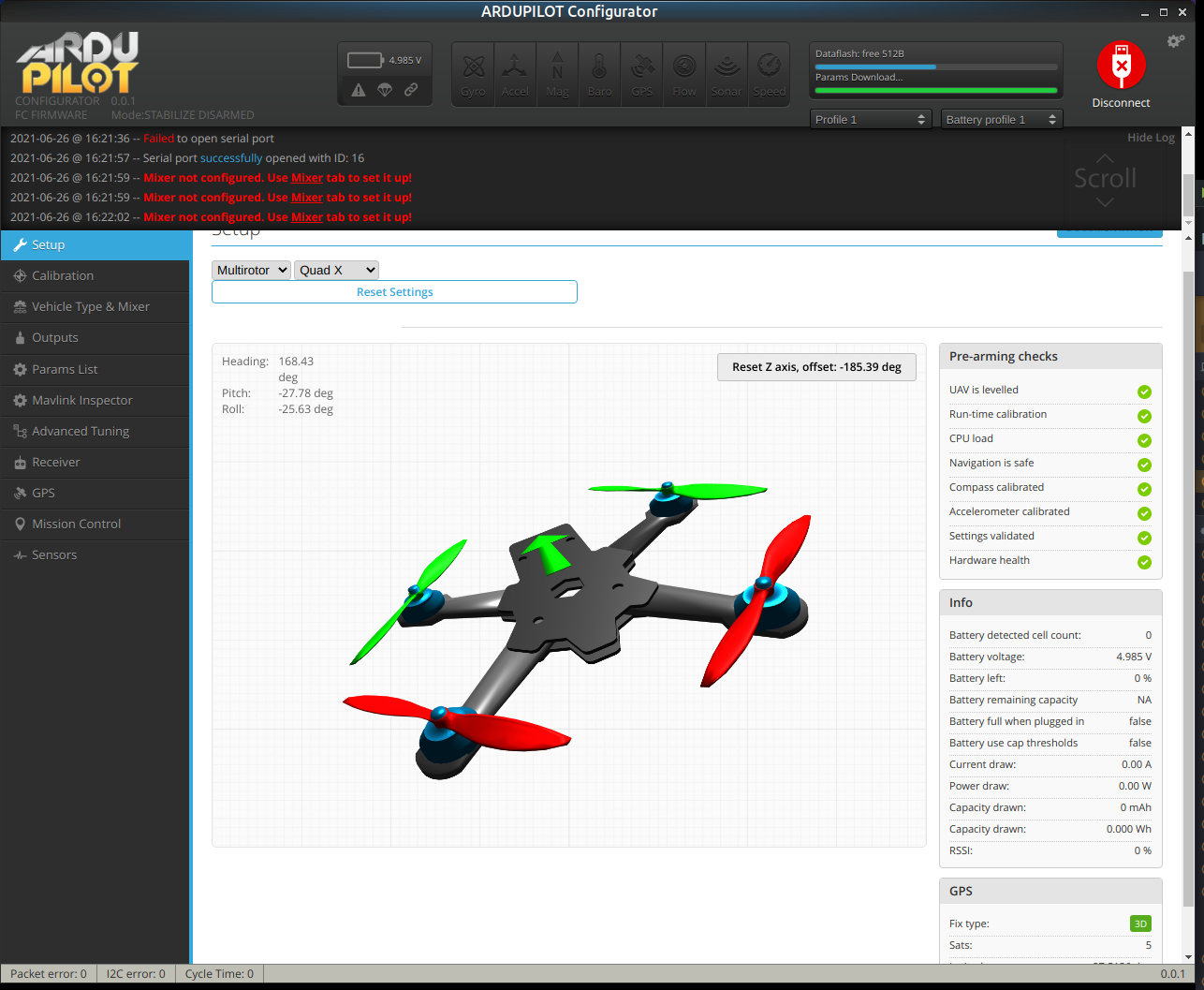The screenshot showcases a website with a predominantly black background. In the top left corner, the logo "ArduPilot" is prominently displayed, with the "O" in "Pilot" designed to resemble a yellow bullseye. Centrally at the top, in small white text, it reads "ArduPilot Configurator." The top right corner features a gray settings icon and a red circular button labeled "Disconnect."

Beneath this header, there's a main section with a white background displaying a colored image of a drone. The drone is equipped with two red-tipped propellers and two lime green-tipped propellers. In the upper right corner of this section, text indicates "Reset Z-axis offset -185.39 DEG." Along the right side of the image, various banners are displayed: a gray banner labeled "Pre-arming checks," followed by another gray banner for "Info" and finally one for "GPS."